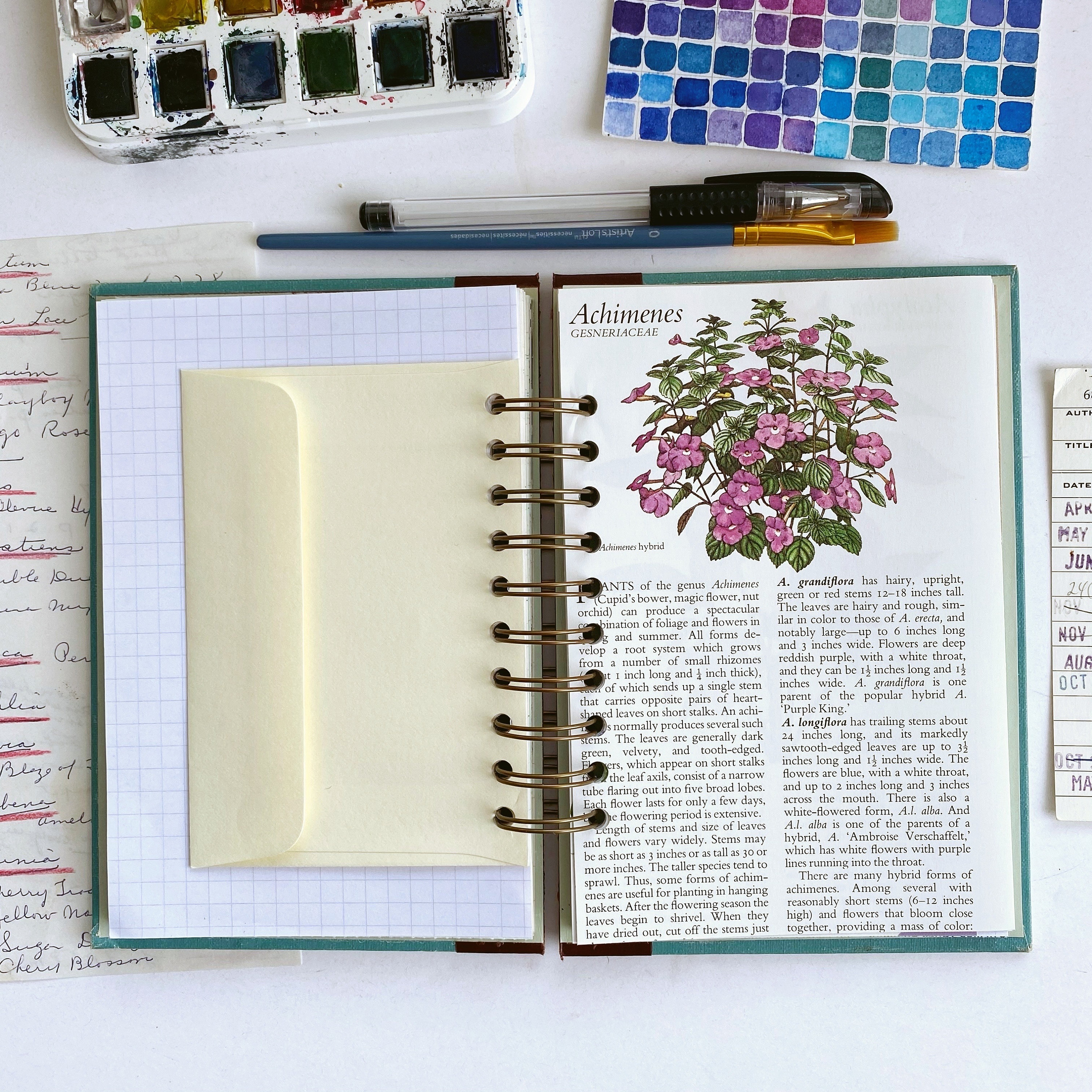The photograph captures a detailed, overhead view of a white desk or table, impeccably arranged as a creative workstation. Central to the square-shaped image is a dark blue scrapbook or notebook, bound by a silver spiral ring with punched holes, revealing a black spine. The open book prominently features an illustration of a purple-flowered plant labeled "Achimenes," alongside a detailed Latin description and accompanying text in two columns. 

On the left page, there’s a cream-colored envelope inserted, overlaying a sheet of grid paper. Above this setup are various art supplies: a black pen with a clear body and a blue pen with a gold cap, a paintbrush, and multiple paint palettes showcasing a gradient of colors from dark to bright. To the right of the book, you can partially see a piece of paper adorned with shades of blue, pink, and purple. 

Additionally, there are scattered handwritten notes under the book on both sides and a possibly partially-visible library card to the left, embellished with dates and underlined names. The entire scene is brightly illuminated, emphasizing the meticulous organization and artistic ambiance of the workspace.